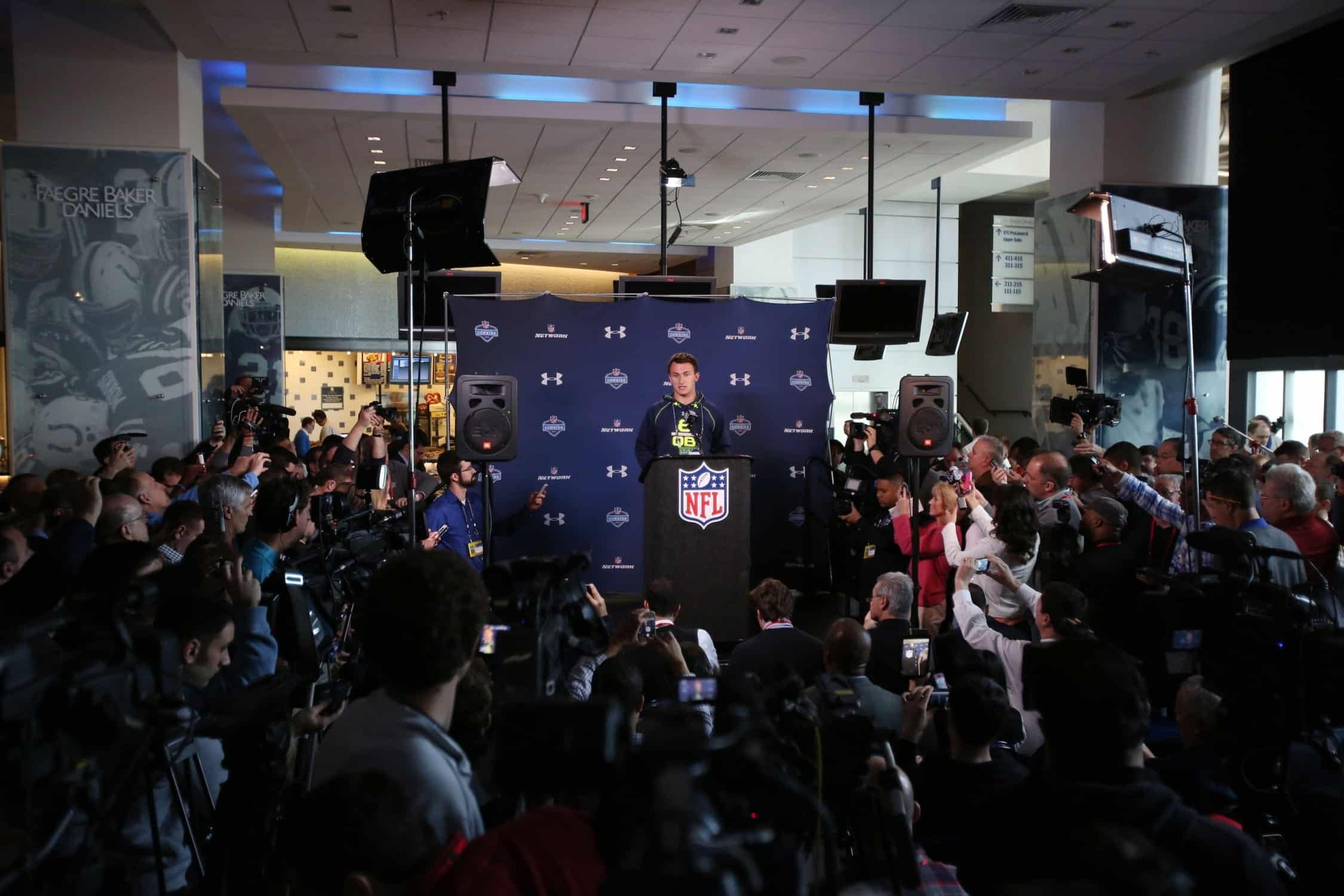The image depicts a detailed and well-lit NFL press conference featuring an athlete, identified as Johnny Manziel, standing behind a black podium emblazoned with the distinctive NFL shield logo. The logo prominently features "NFL" in red letters on a white background, with a blue top section decorated with stars and a white football. Johnny Manziel, a light brown-skinned former football player, is dressed in a black sweatshirt with yellow text across the front.

The backdrop behind Manziel is a blue promotional wall adorned with various logos, including Under Armour and NFL Network. There are also other logos and sponsorships visible, such as the name "Faegre Baker Daniels" on a banner to the left. The area is filled with reporters holding up phones and microphones, eager to record his statements. The setting is brightly illuminated with professional lighting fixtures on stands and hanging from the segmented ceiling, contributing to the image's clear and vibrant colors. The event appears to be taking place indoors, possibly in a store, with some background elements like a pretzel stand faintly visible.